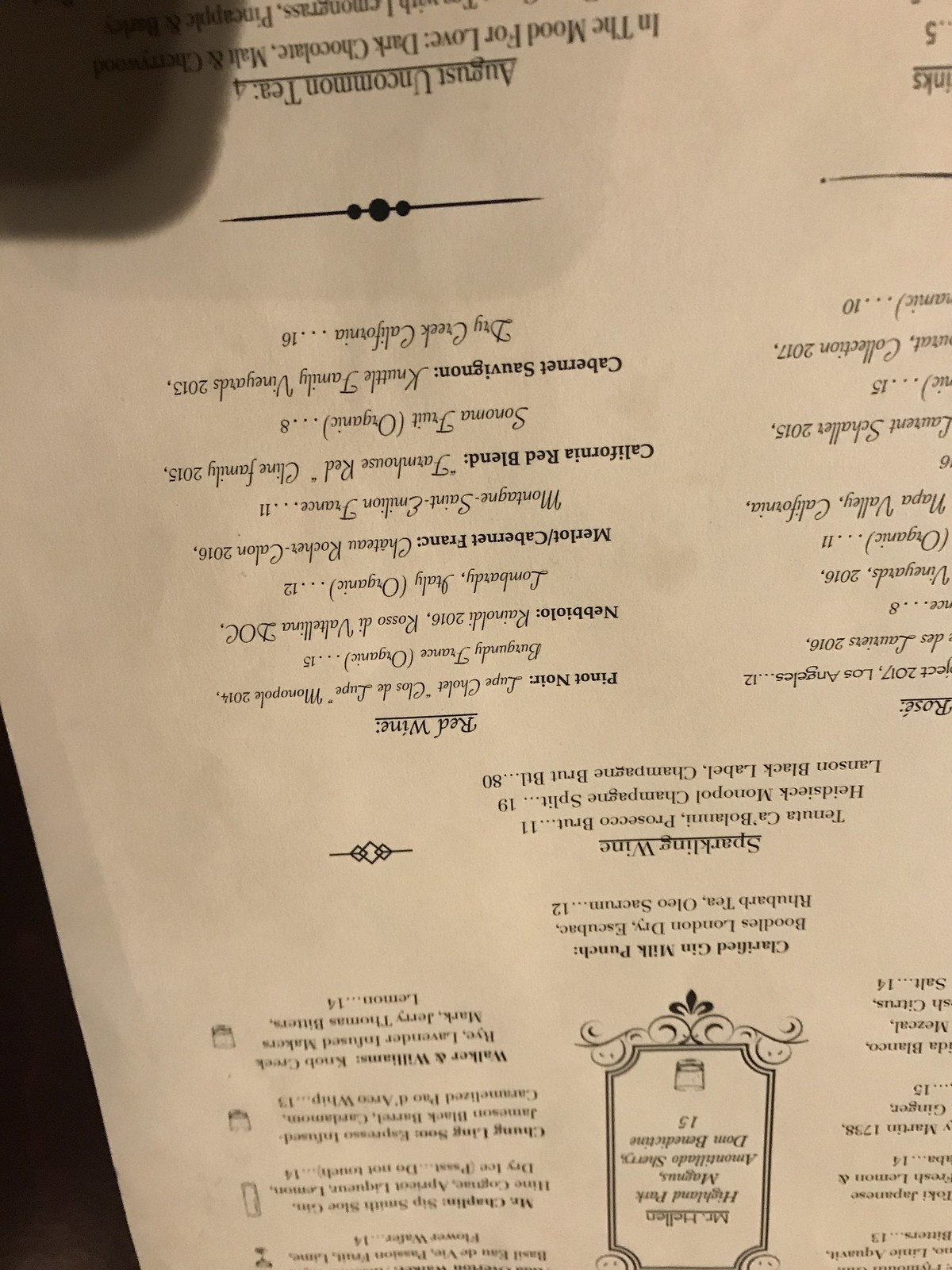An upside-down photograph of a partially visible menu shows intricate cursive writing detailing a variety of offerings, predominantly wines. The menu, slightly angled, leaves a triangular black edge in the bottom left corner of the image, and a phone shadow obfuscates the upper left corner (the menu’s bottom right). The right side of the photograph cuts off part of the left side of the menu, leaving some entries out of view. Sparkling wines and an assortment of foods are hinted at, though specific details remain unreadable due to blurriness near the bottom of the menu, caused by reflective tinting. At the top of the image, clear text reads "August Uncommon Tea," followed by slightly obscured writings, "In the Mood for Love Dark Chocolate Malt," with the rest hidden by a shadow.